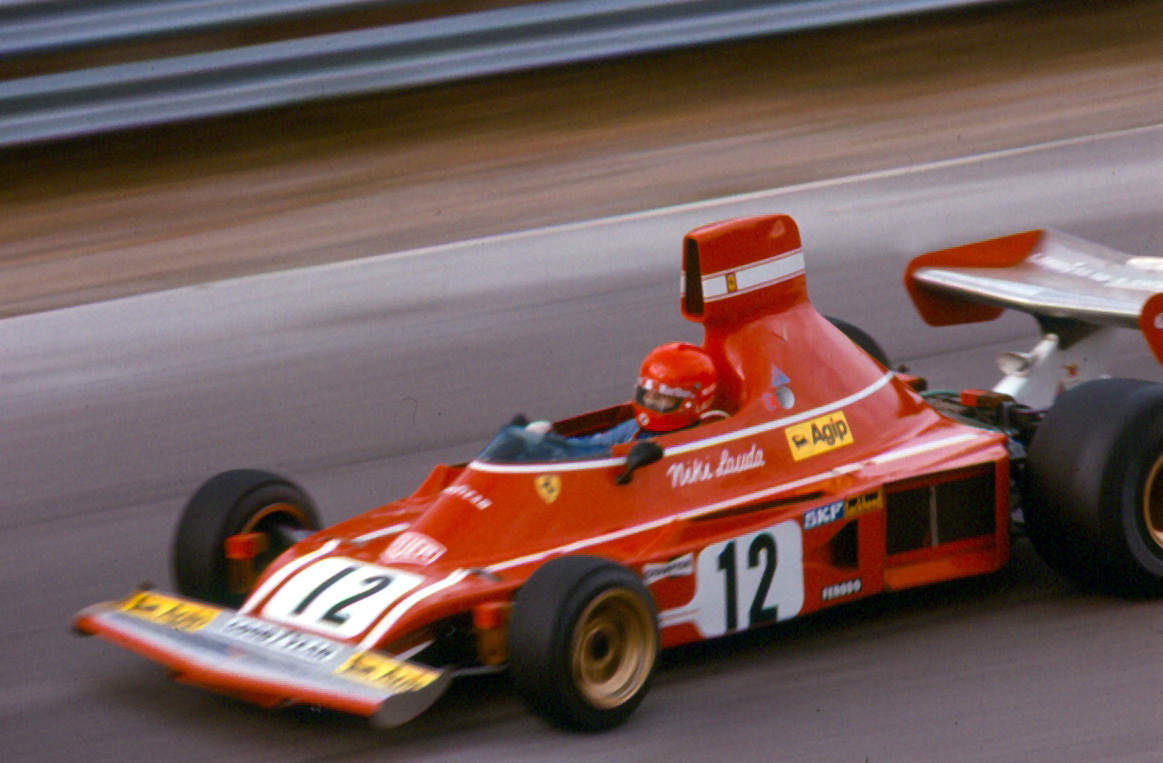This image captures Formula 1 driver Niki Lauda in the midst of a high-speed race, piloting a distinctively classic red Ferrari. The race car, marked with the number 12 in bold black text within a white box, features several notable sponsor logos, including Nike, Tag Heuer, Goodyear, AGIP, and Lada, though some texts are harder to discern. The car's design, with its large rear wheels and pronounced spoiler, suggests it hails from a bygone era, quite different from modern F1 machines. Lauda, wearing a red helmet, appears focused and intense, though his face remains obscured. The image, likely taken by a professional photographer, perfectly captures the dynamic motion of the event with the background rendered as streaked blurs, enhancing the sensation of speed. The car's intricate colors include red, black, white, silver, gray, orange, yellow, tan, and various shades of brown, adding a rich, detailed palette to the scene.